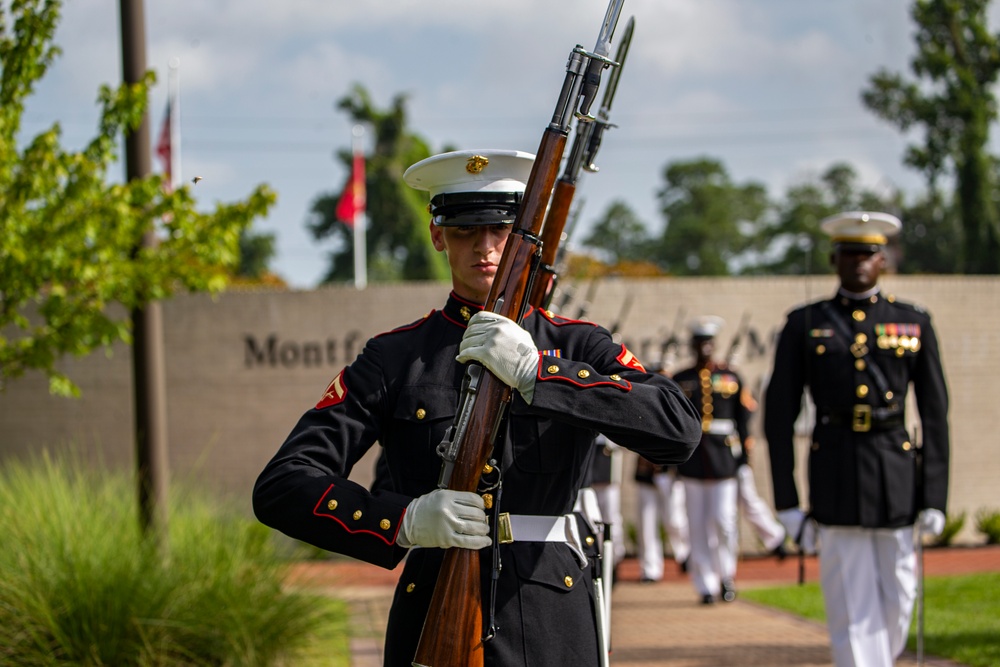The photograph captures a meticulously detailed scene of U.S. Marines engaged in what appears to be a parade or ceremony. Dominating the foreground is a white Marine, looking directly at the camera with a serious expression. He’s dressed in the traditional dark blue dress uniform adorned with several gold buttons—three on each sleeve and more along the front—complemented by red and yellow patches. His white belt, accentuated by a gold belt buckle, stands out against the dark uniform. 

On his head, he sports a white cap with a black brim and a distinguished gold medallion at the center. His gloved hands hold a brown rifle with a fixed bayonet, the left hand gripping the butt and the right securing the barrel. The rifle is held in a position suggesting readiness and formality. 

In the midground, another Marine, an African American, appears slightly blurred but clearly wears the same uniform. This second Marine displays several medals on his chest, indicating a higher rank. His arms hang straight at his sides as he marches, contributing to an overall impression of disciplined movement.

The background is a bit unfocused, revealing more Marines who seem to be participating in the same event. They march in unison against the backdrop of a large brick wall bearing partially obscured black writing that starts with "M-O-N-T-F." The scene also features a tall grassy plant and the hint of a tree in the upper left corner. Two flags can be identified near the concrete wall, one of which is undoubtedly the American flag, while the other remains partially obscured and red in color.

Overall, the photograph encapsulates the precision, formality, and unity emblematic of a U.S. Marine Corps event, set against an outdoor backdrop that adds context to the ceremony’s location.